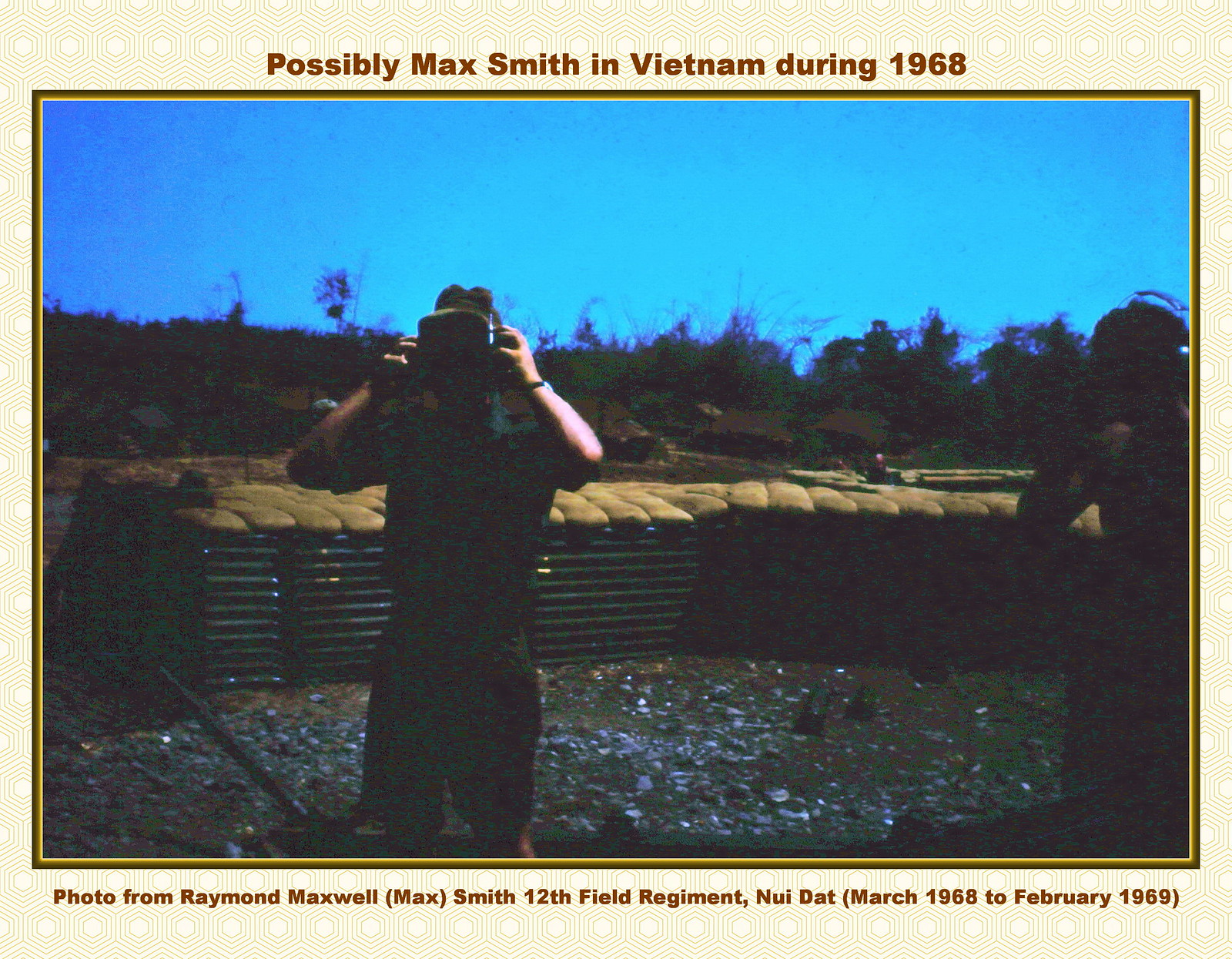This is an extremely faded full-color photograph framed with a brown and white hexagonal pattern border, featuring an additional dark brown and gold border. The image is horizontally aligned, capturing a clear blue, cloudless sky over a military base likely in Nui Dat, Vietnam, during 1968. At the top, brown text reads "Possibly Max Smith in Vietnam during 1968," while at the bottom, the caption says, "Photo from Raymond Maxwell (Max) Smith, 12th Field Regiment, Nui Dat, March 1968 to February 1969."

The scene shows two indistinguishable men due to shadowing, standing amidst a sandy, rocky terrain fortified with stacked sandbags. The man closer to the center is holding a large camera in front of his face, wearing short sleeves, a watch, and possibly pulling off a helmet. The man on the far right appears to be wearing a blue hat, and trees or plants are visible in the background. Despite their dark uniforms, the overall impression suggests they are stationed in a foxhole or trench setting typical of military defense operations.